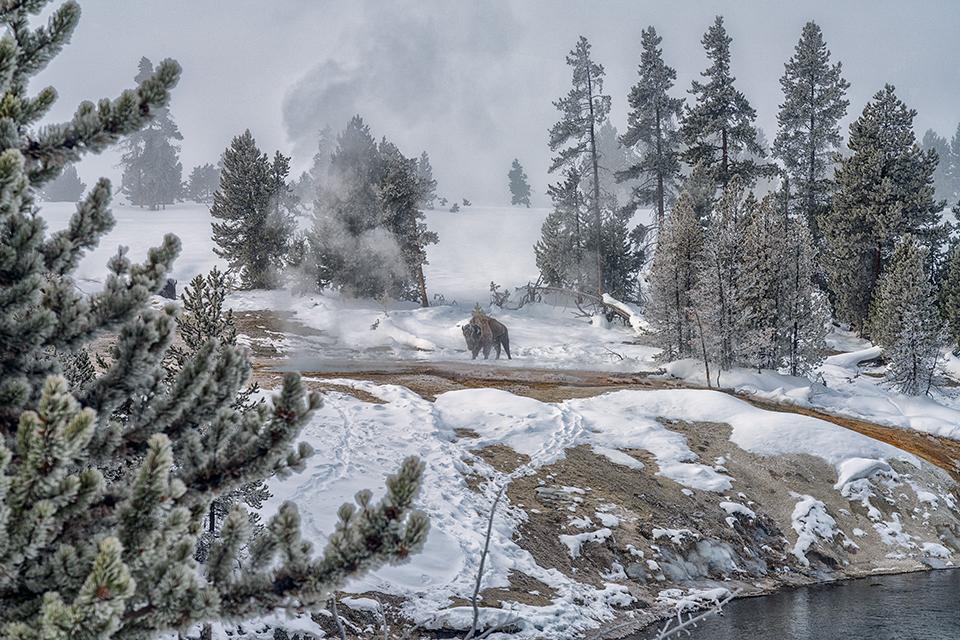In this evocative winter scene, a lone buffalo stands stoically at the center, set against a backdrop of snow-covered ground and a gray, overcast sky. The buffalo, with its brown and black fur, is positioned on the bank of a waterway, possibly a lake or river, where the snow has started to melt, revealing patches of dirt and rocks. Surrounding this central figure, snow-laden pine trees and slightly barren ones create clustered arrangements that evoke the look of classic Christmas trees. Mist rises subtly in the left portion of the image, adding to the chilly atmosphere. The somber, color-muted landscape stretches into the distance, where more trees punctuate the snowy field, and the horizon blends seamlessly into the cloudy sky. This photograph vividly captures the serene stillness and stark beauty of a winter landscape.